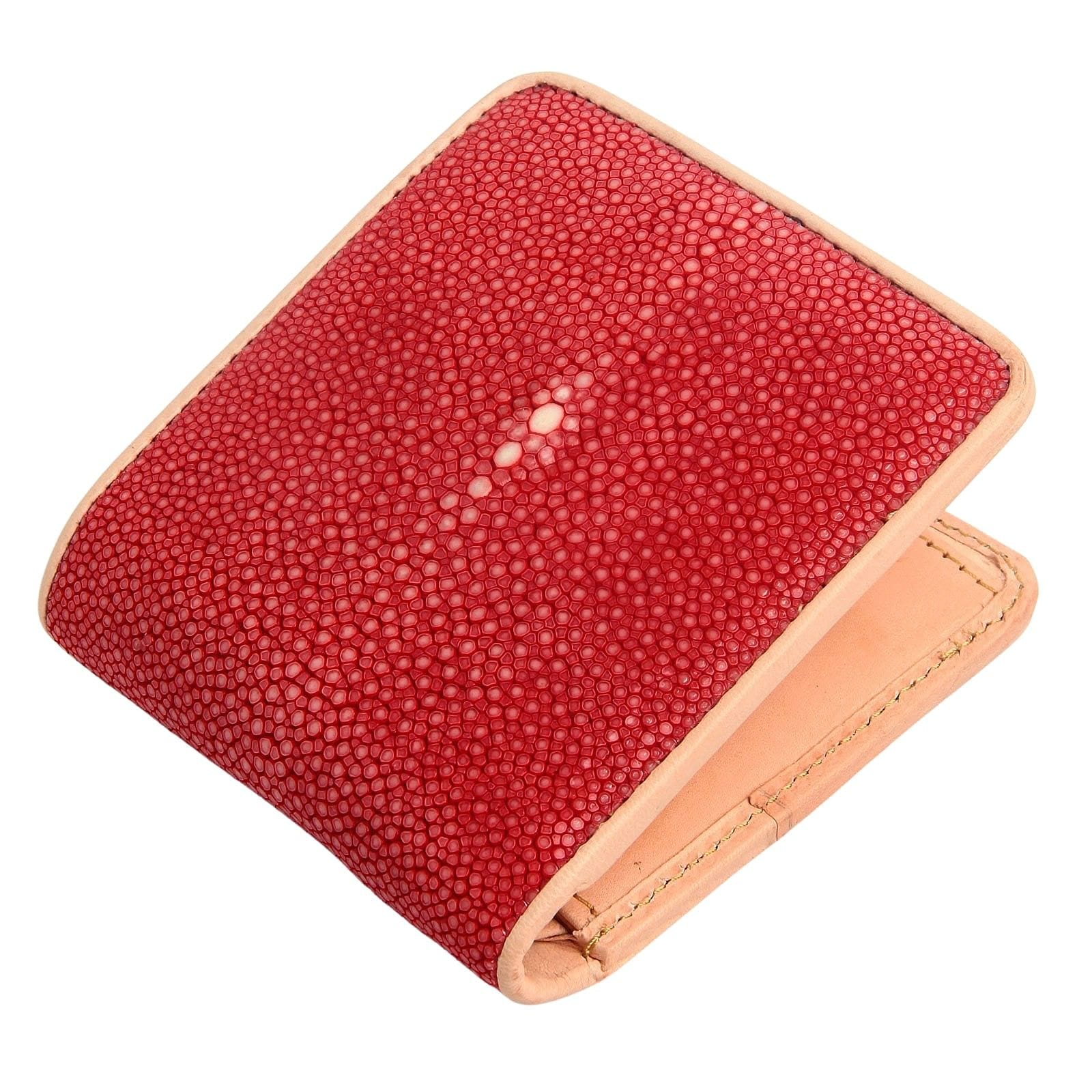The image depicts a stylish women's bi-fold wallet. The exterior is predominantly red, accentuated with a border of peach or salmon color. The red surface is dotted with a white bubbly texture, providing a unique pattern. Intricate stitches along the edges highlight the craftsmanship. The wallet, which folds once at the center, reveals glimpses of its interior, showcasing a pink hue that complements the outer design. The interior also appears to have a functional pocket or possibly a zipper section aligning with the curve where the wallet folds. The background of the image is stark white, emphasizing the wallet's colors and details, making it a clean and professional stock photo.